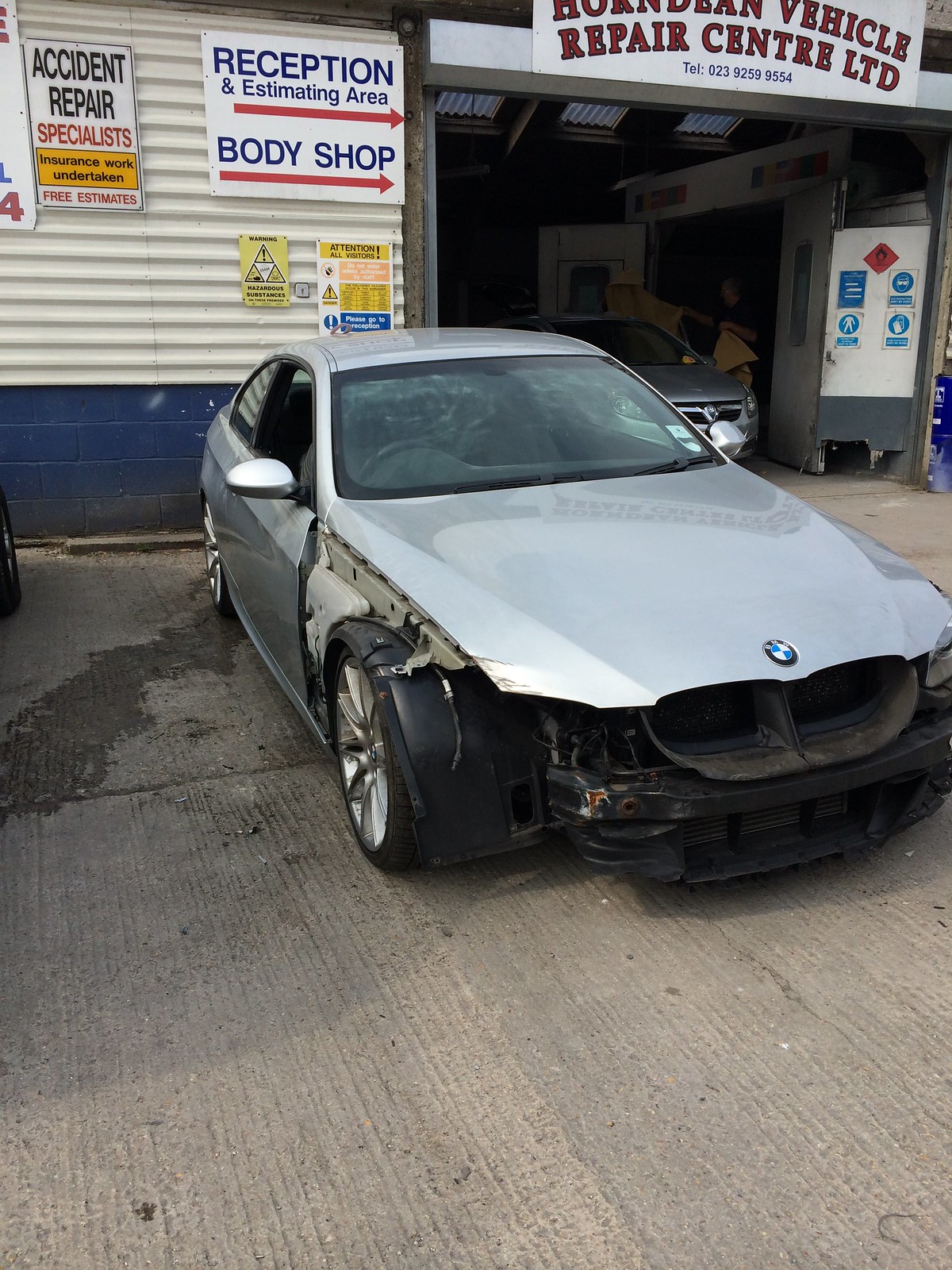The image depicts the exterior of the Hornedean Vehicle Repair Center Limited. In the foreground, a silver BMW coupe, facing the viewer, is prominently parked in front of the garage. The BMW is severely damaged, missing its entire front grille, front bumper, and both headlights. Additionally, there is a noticeable absence of the front right quarter panel (fender) and possible underlying components. The hood shows damage on the driver's right side. Above the garage door, signage reads "Repair Center Limited," though it is somewhat obscured. To the left of the BMW on the wall are signs advertising "Accident Repair Specialists," "Insurance Work Undertaken," and "Free Estimates." Adjacent to these, another sign with red arrows points towards the "Reception and Estimating Area" and "Body Shop." In the background inside the garage, another silver vehicle is visible, indicating it is currently being worked on. The ground in front of the repair center is concrete.